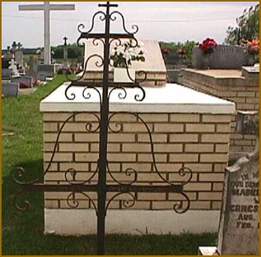In the cemetery photo, the focal point is an ornate steel cross situated in front of a tomb. The cross is decorated with intricate swirly designs and forms resembling waves or ribbons, creating a bell shape on each level. The tomb itself has a white lid, yellow brick sides, and a white base. Surrounding this central tomb are various other gravestones and crosses, including a prominent larger white cross in the background to the left. A black gate with some wires can be seen at the front, adding to the solemn atmosphere of the cemetery. Among the graves, flowers are visible on another tomb, contributing a touch of color to the scene. The image captures a lush green lawn and scattered trees, suggesting a summertime setting, despite the somewhat hazy, gray sky. The overall ambiance is serene yet somber, accentuated by the meticulously detailed cross and the variety of tombstones that populate the background.